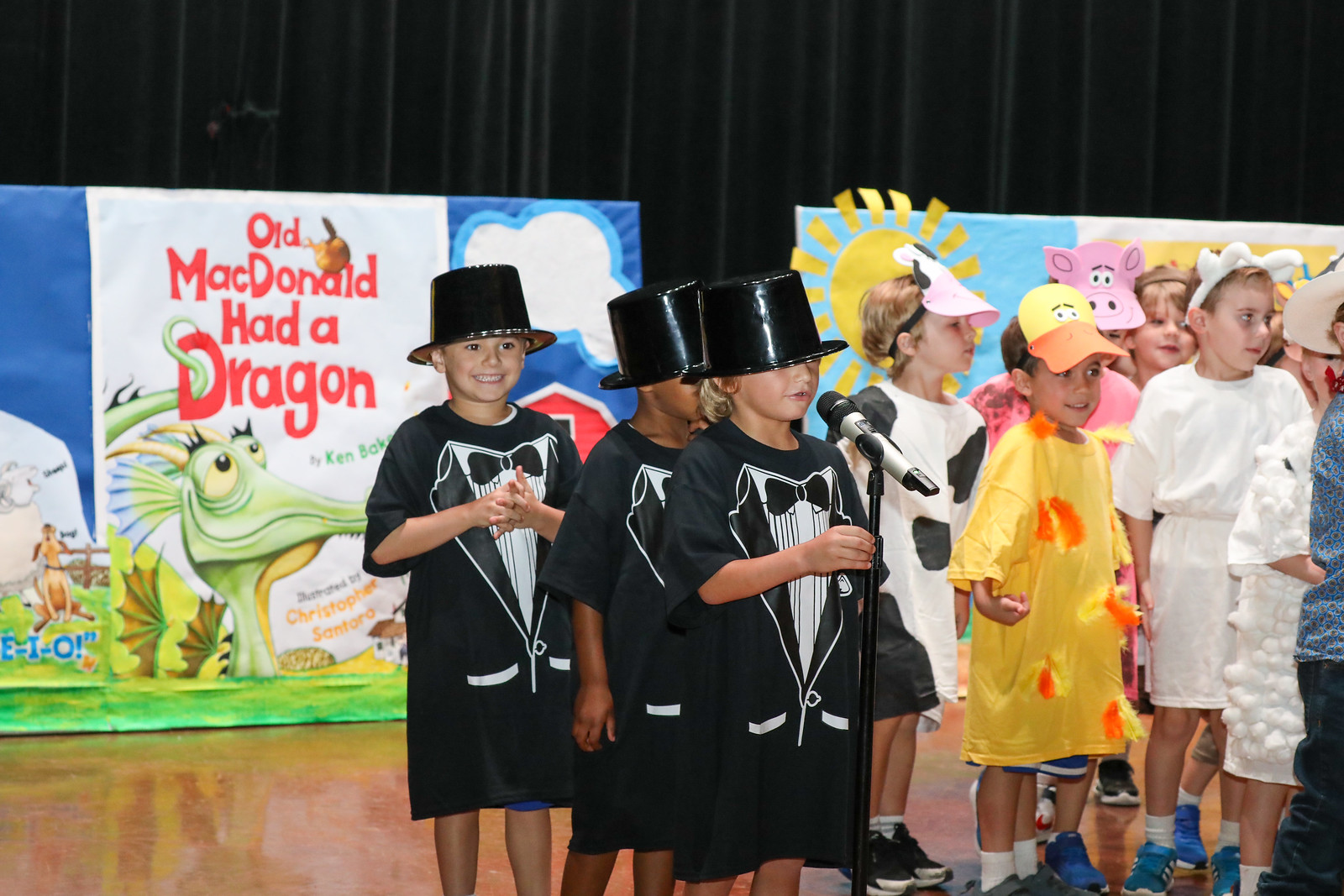This detailed photograph captures a scene from a children's play titled "Old MacDonald Had a Dragon." On a wooden stage with a black curtain backdrop, three boys stand in a line at center stage, each wearing costume tuxedo shirts and black top hats. The boy in front speaks into a silver microphone, while the other two stand behind him. 

To the right, a group of children dressed in various animal costumes adds vibrant color and charm to the scene. Among them is a girl dressed as a cow, a child in a pink costume, another in yellow, and others in white, each adorned with accessories such as hats, masks, and bunny ears, representing different barn animals like ducks, pigs, and sheep. 

The background features large paper posters, one prominently displaying the play's title, "Old MacDonald Had a Dragon," alongside illustrations including a friendly, smiling green dragon with big eyes, set against a backdrop of blue skies and clouds. This charming and lively stage scene perfectly encapsulates the whimsical and joyful essence of a children's performance.